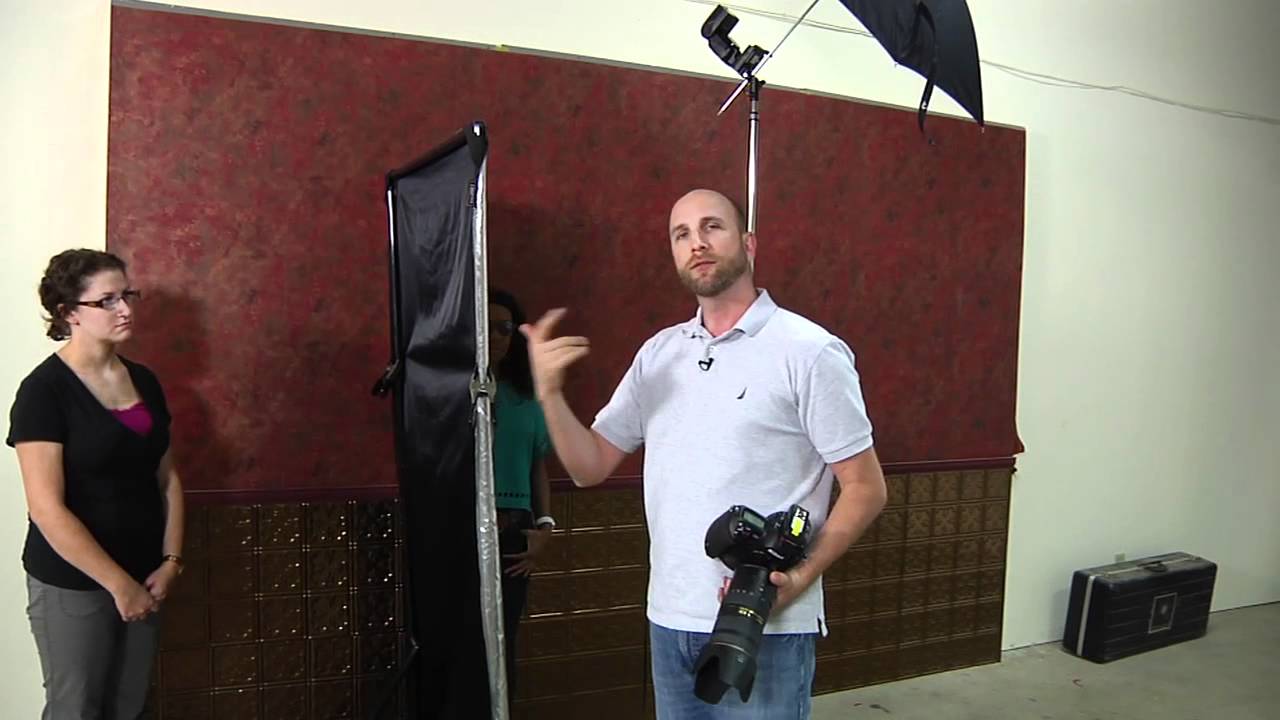In the center of this horizontal color photograph, a professional photographer, dressed in jeans and a short-sleeve collared shirt, possibly a Ralph Lauren polo, is engaged in conversation. He is gesturing with his right hand raised while holding a camera with a very long lens in his left hand. The man, who is balding with a mustache and a close-cropped beard, stands near a black background screen, likely used to enhance the clarity of his photographs. 

To his left, a woman in a black shirt layered over a purple tank top and gray pants, with black hair and glasses, listens intently. Another woman, wearing a green shirt, is partially visible against the wall. Above the photographer, and attached to a long pole, is a black umbrella, typical of studio lighting setups. Additionally, a black case rests along the wall, possibly containing more photography equipment. This image captures an ongoing photo shoot, offering a glimpse into the dynamic interaction between the photographer and his subjects or assistants.